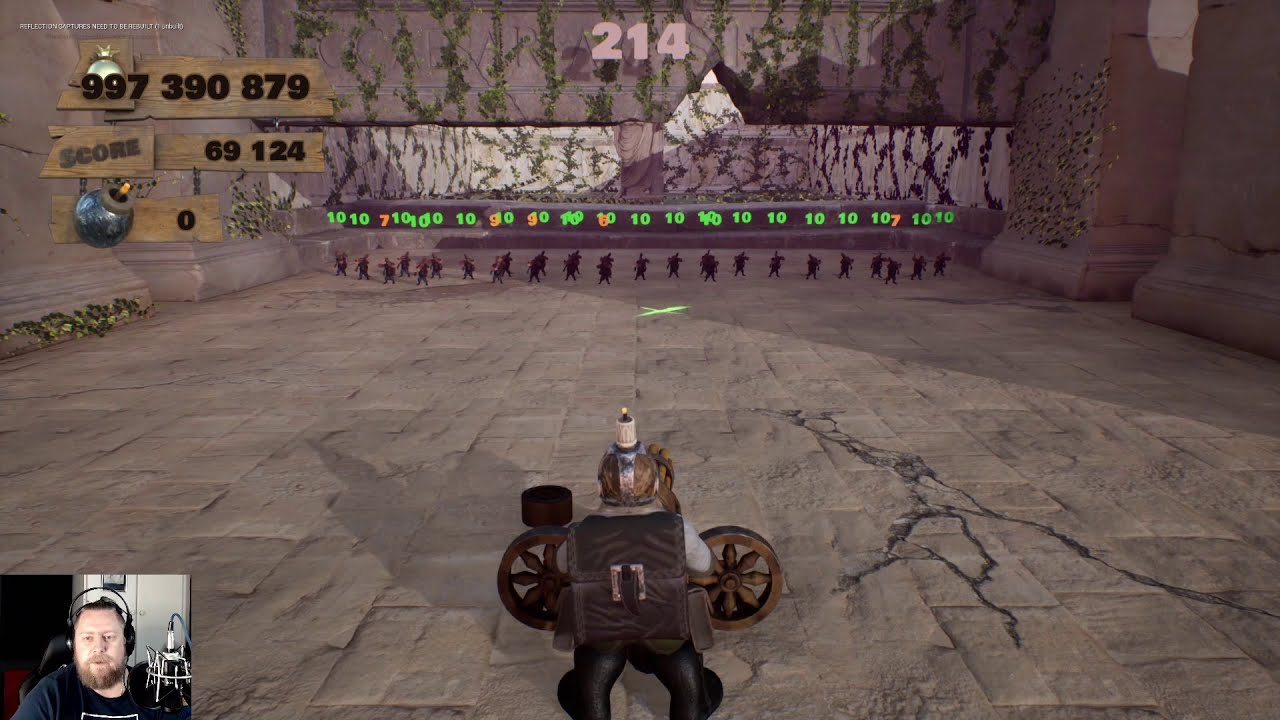The image is a detailed screenshot from a video game live stream, showcasing both the game environment and the player's webcam feed. In the bottom left-hand corner, a rectangular inset displays a young, heavyset white man with a full light brown beard and black headphones, sitting in a black gaming chair. He wears a dark t-shirt with a white logo and appears to be streaming his gameplay live, likely from a white room filled with electronic equipment.

The game screen itself presents a third-person view of the player's character in a large weathered stone room or courtyard. The floor, made of grey stone tiles, shows prominent cracks spreading outwards, suggesting it is falling apart in places. The character is equipped with an elaborate backpack and has wheels on either side of his body, wearing black pants. A peculiar flamethrower protrudes from his helmet.

The far wall of the room features vines and a multitude of neon green and orange numbers. There is also a swarm of small black figures, possibly enemies, bearing numbers like 10, 7, 9, and 8, indicating a combat scenario. The upper left corner of the screen displays various stats in brown boxes: a score of 69,124, a sequence of numbers 997-390-879, and another box showing a bomb count of zero. The prominently visible number 214 is also displayed near the top part of the image.